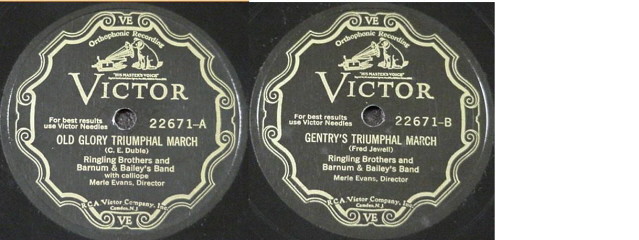The image displays a close-up of two antique Victor black vinyl record labels, showcasing their intricate designs and details. Each label features a dark gray background with text and images in light tan or gold. Prominently at the top, one can see "VE" and "Orthophonic Recording" followed by the iconic RCA Victor logo of a dog, Nipper, attentively listening to a Victrola's horn. The label on the left is marked "22671-A" and titled "Old Glory, Triumphal March" performed by Ringling Brothers and Barnum & Bailey's Band with a Calliope, under the direction of Merrill Evans. The right label, "22671-B," titled "Gentry's Triumphal March" by Fred Jewell, is similarly performed by the Ringling Brothers and Barnum & Bailey's Band, directed by Merrill Evans. Both labels feature decorative borders and highlight that they are best played with Victor needles. They also include the imprint "RCA Victor Company Incorporated, Camden, New Jersey" at the bottom, emphasizing their vintage status.